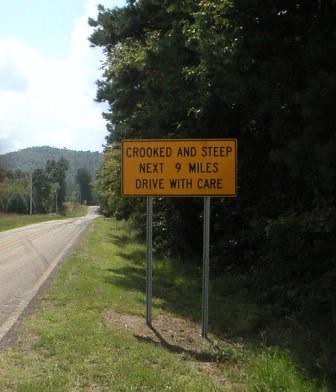In this photo, a paved road stretches diagonally from the bottom left corner toward the center, bordered by a white painted line on its visible right side. Beside the road sits a prominent orange road sign supported by two metal poles. The sign reads, "Crooked and steep. Next nine miles drive with care," and is positioned within a grassy area dotted with small stones and a dirt patch. To the right, a line of tall, leafy bushes stands lush and green. In the background, under a canopy of blue sky adorned with wispy clouds, a distant mountain or hill rises majestically, flanked by tall trees that mirror the greenery of the foreground.